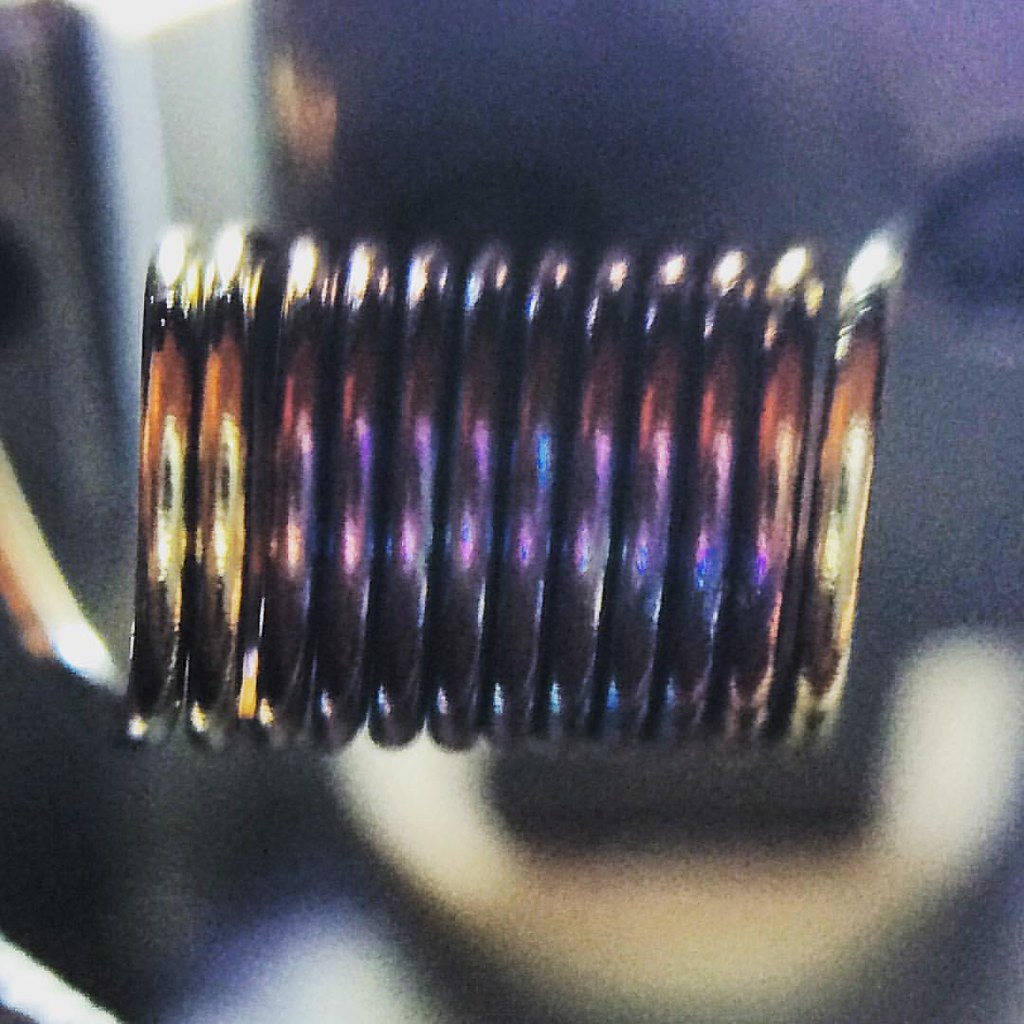The image features a close-up of what appears to be a set of round, metal rings or a tightly wound coil. The rings seem to be predominantly gold, but they are extremely shiny and their reflective surfaces pick up various colors from their surroundings, including purple, orange, and blue, creating a rainbow-like effect. The rings or coils are moderately sized, not overly large, and it is evident that they are not connected, with visible spaces in between them. The background is heavily blurred, with vague, indistinct shapes that include shades of gray, cream, and black, making it difficult to discern any specific objects. The blurred background adds to the focus on the metallic rings or coil in the foreground, which dominate approximately half of the image.